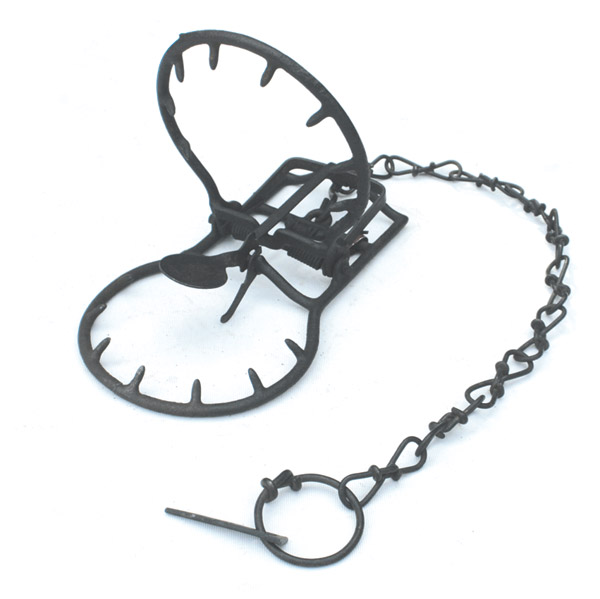In this detailed photograph, the white background starkly contrasts with a prominent animal trap positioned towards the left side, facing left. The trap features circular top and bottom sections equipped with menacing, pointed metal teeth designed to snap shut when the central trigger mechanism is activated by pressure. At the back of the trap, a mechanism housed in a square structure connects to a grayish-black chain. This chain curves around the right side of the frame before looping back under the main body of the trap on the left. At its end, the chain attaches to a large, round metal ring, through which a metal stick extends, possibly serving as an anchoring spike. The entire trap showcases a black matte, rusty metal finish, creating an impression of both age and functionality.